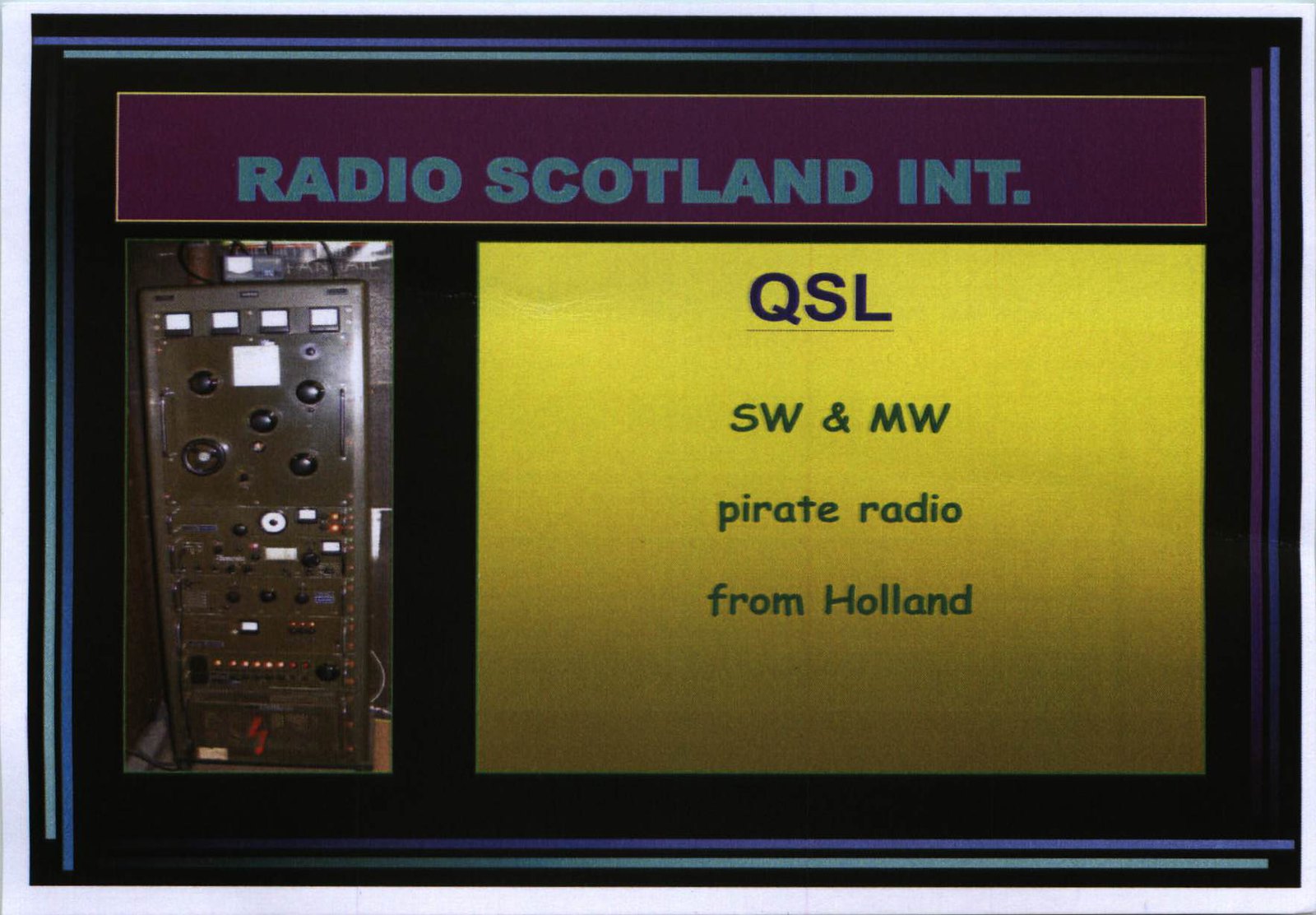The image showcases a display, possibly set behind glass, featuring a magazine or newspaper layout. Dominating the top portion is a dark red banner with a thin yellow border, adorned with bold, blue block letters reading "Radio Scotland INT." Below that, to the right, a yellow placard contains black text stating "QSL," followed by "SW and MW," and "Pirate Radio from Holland." To the left side of the display, there's a detailed picture of old pirate radio equipment, featuring a vertically-oriented, metallic radio station setup. This machine is black, tall, and rectangular, adorned with numerous round and square buttons in black and white, as well as several gauges and jack openings. The background is primarily black, framed by a white border that includes thin strips of blue, green, magenta, and purple along the sides. This display appears to be a historical representation of pirate radio broadcasting equipment used by Radio Scotland International.